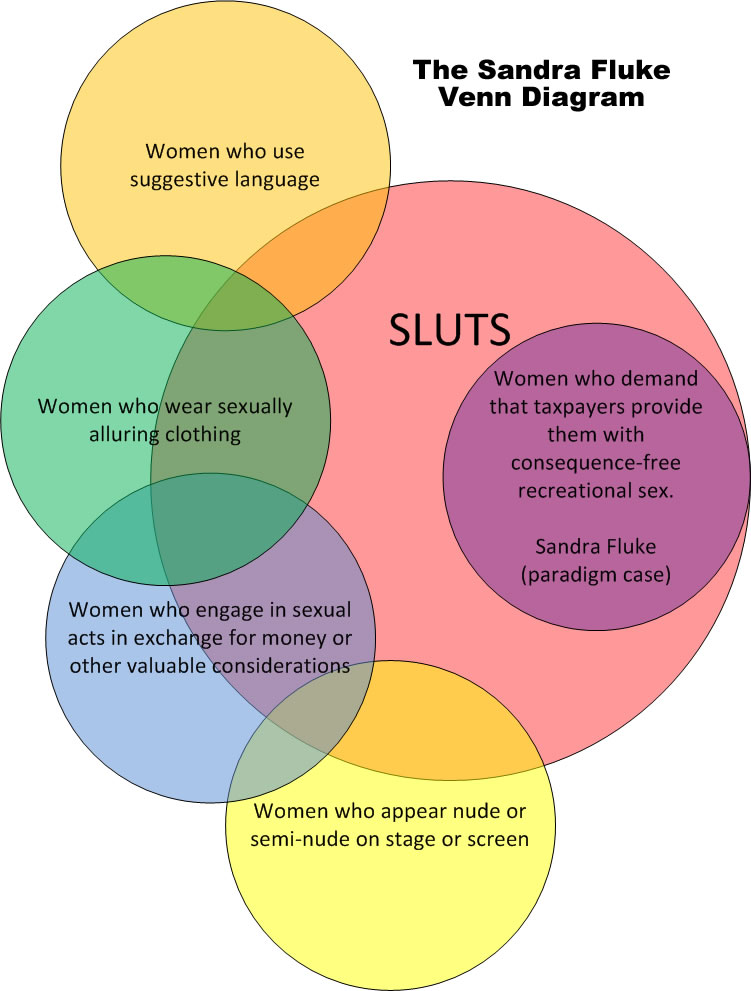The image is a Venn diagram titled "The Sandra Fluke Venn Diagram" in bold black letters at the top. Central to the diagram is a large peach-colored circle labeled "Sluts." Encompassed entirely within this main circle is a lavender circle that reads, "Women who demand that taxpayers provide them with consequence-free recreational sex, Sandra Fluke (paradigm case)," which seems to be a direct jab at her. Surrounding the central peach circle and partially overlapping it are several other smaller circles in various colors: a yellow circle labeled "Women who use suggestive language," a green circle for "Women who wear sexually alluring clothing," a blue circle for "Women who engage in sexual acts in exchange for money or other valuable considerations," and another yellow circle labeled "Women who appear nude or semi-nude on stage or screen." The arrangement and coloring — peach, purple, green, yellow, and blue — visually depict how different behaviors and attributes are associated and overlapping within the category pejoratively labeled as "sluts."